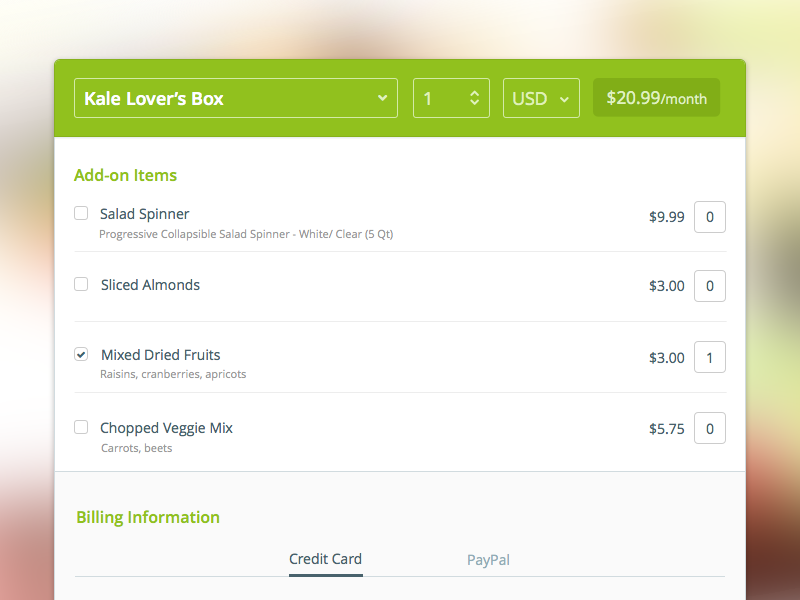This section of the website provides options for purchasing a subscription box. 

At the top, there's a green rectangular dropdown text box with white lettering that reads "Kale Lovers Box". To the right of this, there is a dropdown tab labeled with the number "1", indicating the quantity. Another dropdown tab next to it provides various selectable options. 

Adjacent to these dropdown boxes, there is a darker green box displaying the price "$20.99 per month". Below this pricing information, a white box is available for selecting add-on items. On the right side, you see a list of items with checkboxes to their right, allowing for multiple selections. 

Each item is detailed, showing its name, description, and price. In this example, only the third option, "Mixed Dry Nuts", has been selected. It is described as containing raisins, cranberries, and apricots, with a price of $3 for one order.

Below the add-on items list, there is a section for billing information that offers payment options via credit card or PayPal.